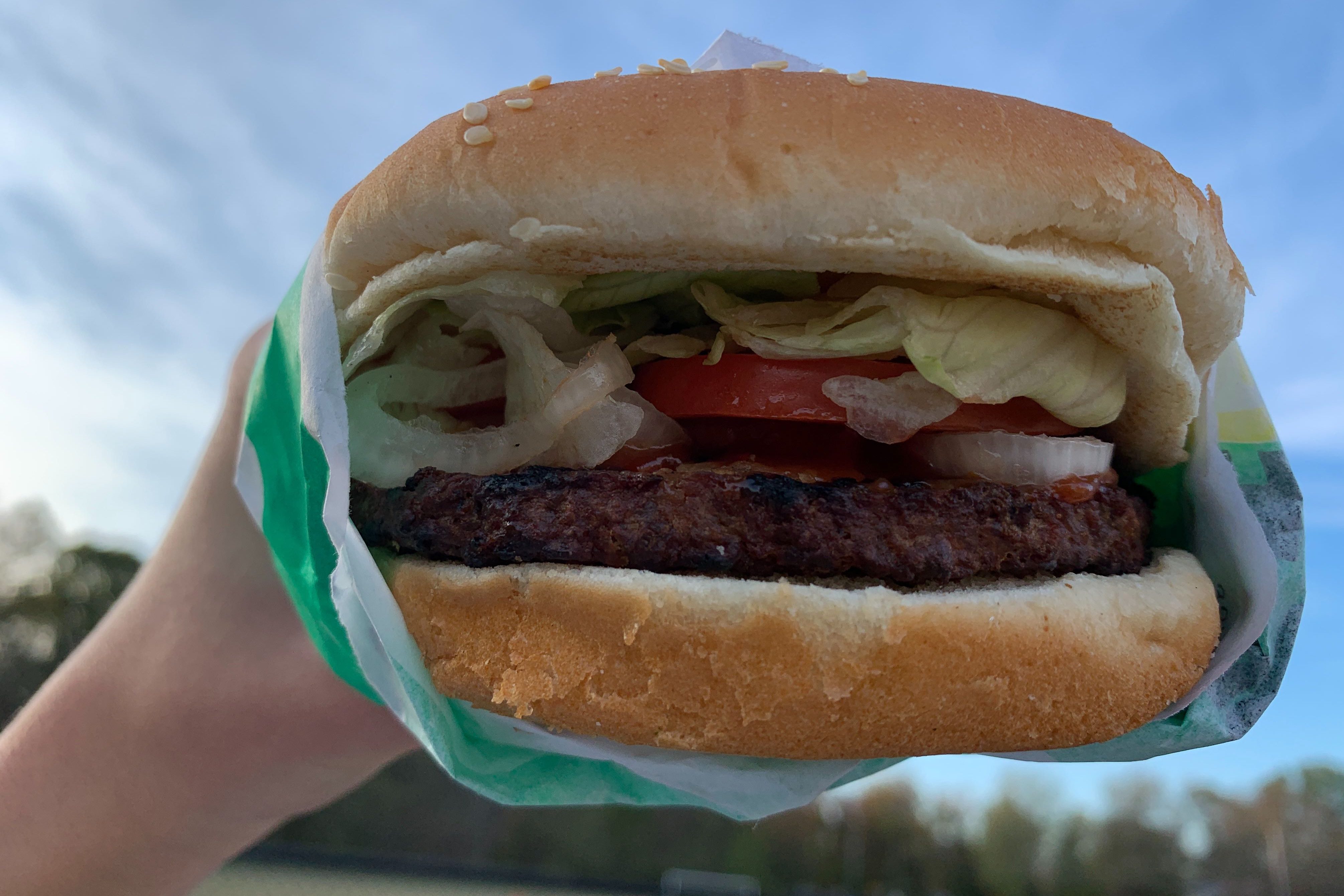This detailed photograph, rectangular in landscape, features a large cheeseburger prominently held up by a Caucasian left hand. Despite the close-up shot, the burger's significant size is evident, overshadowing the blurred background. The lightly tanned bun, sparsely dotted with sesame seeds, crowns the burger atop crisp layers of lettuce, tomato slices, and onions. A single juicy patty sits comfortably on the lower bun layered with condiments like ketchup. The burger is partially wrapped in a white, green, and yellow striped fast-food wrapper, characteristic of many takeaway joints. The backdrop showcases a bright, sunny day with a clear blue sky occupying the majority of the frame, interspersed with light clouds and hints of green foliage and a building towards the left. The setting creates an impression of a casual outdoor scene, further emphasizing the burger's allure.